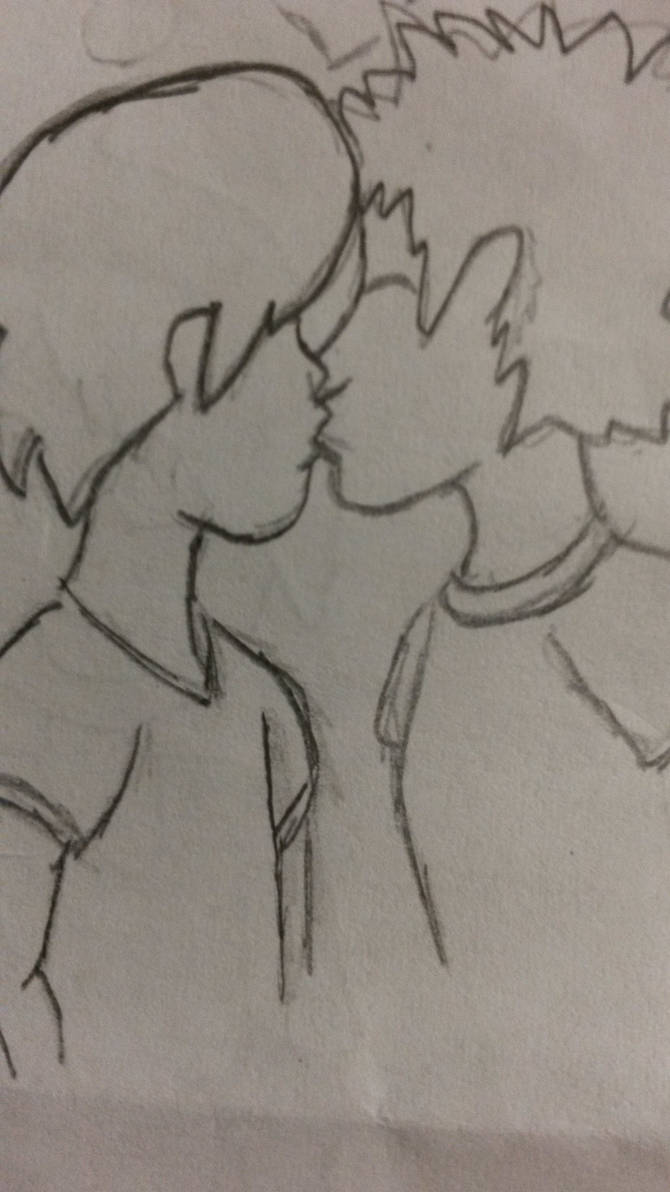The image is a photograph of a sketch drawn on a white piece of paper, which shows various wrinkles and faded lines from previous, likely erased, sketches. This hand-drawn picture, rendered in a pencil-like material, features two young male figures kissing. The lines of the drawing appear jagged and grainy in some areas. The character on the left is facing right, wearing a v-neck short-sleeved shirt, with soft, combed-back hair. The figure on the right faces left, clad in a crew neck collared short-sleeved t-shirt, and has spiky hair. Both characters are only visible from the waist up. Their lips are linked, and their noses are touching in the image. The sketch is simple, with more detail around the necklines and sleeves of their shirts rather than their faces. The figures are rather thin, with no defining female characteristics, suggesting they are both male. Additionally, there are visible erase marks throughout the image, emphasizing its rough, personal, and somewhat unfinished nature.